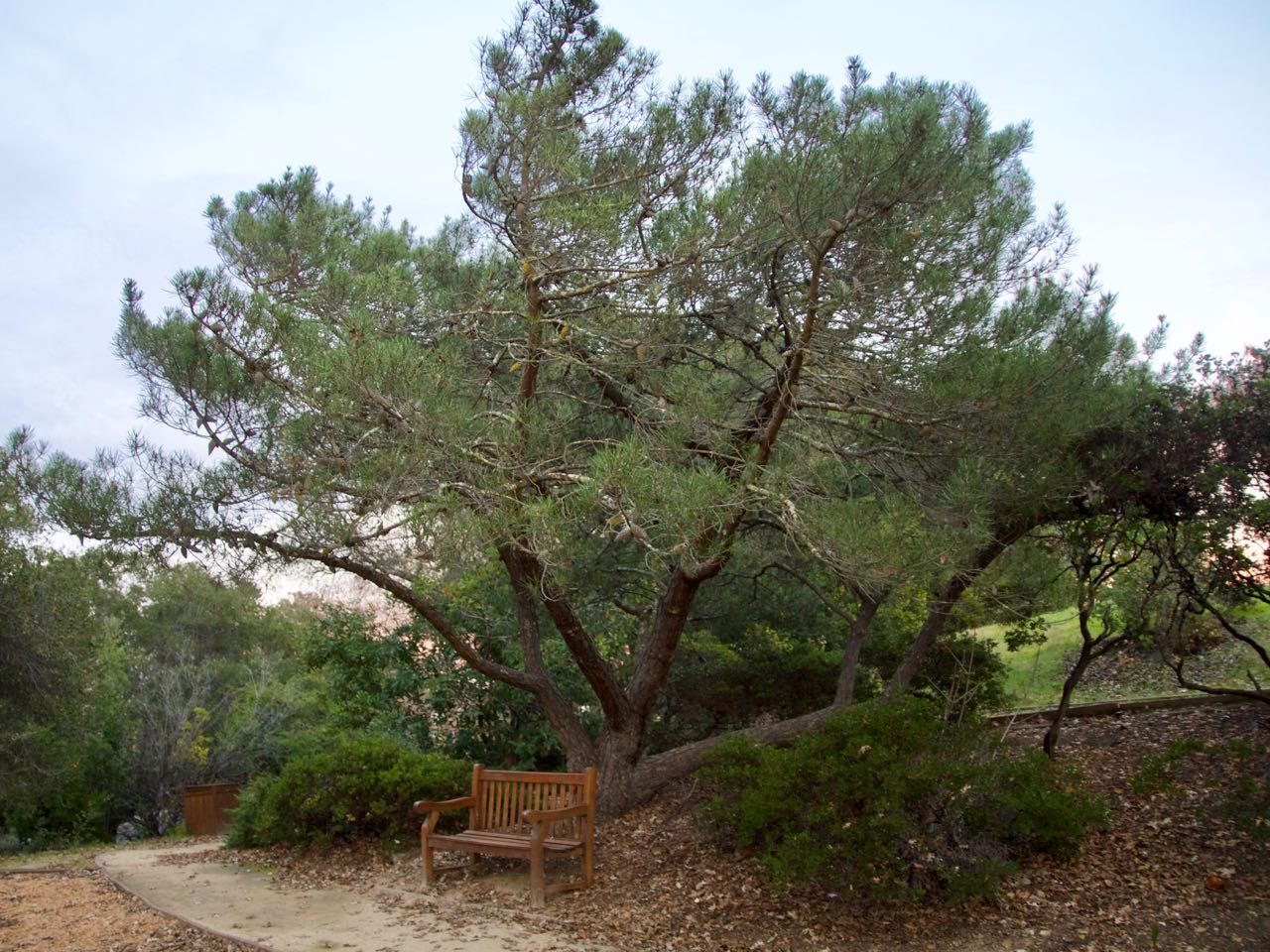The image captures a serene park scene under a clear blue sky with faint white clouds. At the center, a light brown wooden bench, well-maintained and not overly weathered, is angled to face the lower left corner of the picture. It sits adjacent to a paved pathway bordered by mulch, presumably for walking. The bench is nestled under a sprawling, medium-sized evergreen tree with multiple trunks branching outwards and upwards in varying directions, displaying thick, gray bark and needle-like foliage. The ground around the bench features a mulched area mixed with scattered leaves and debris. Several bushes are situated in the lower right corner. To the left of the path, there is a visible area with mulch transitioning into a grassy hillside that ascends gently, contributing to the natural beauty of the park. A wooden structure, possibly a box, is discernible on the far left side of the photo. The scene conveys a peaceful outdoor setting, perfect for relaxation and enjoyment of nature.